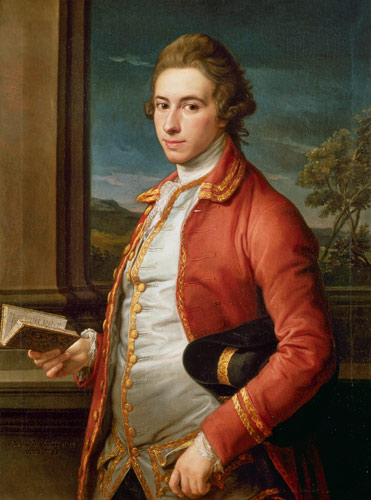This is a detailed painting of a distinguished soldier from an older era, reminiscent of British Revolutionary times. He is adorned in a striking red coat, embellished with intricate gold trimmings along the collar, down the front, and near the cuffs. Underneath, he wears a shiny white shirt with matching gold trimmings and ornate golden buttons. The soldier holds an open book in his right hand, suggesting he paused reading to pose for the portrait; it might be the Bible or another book. Tucked under his left elbow is a black hat with elegant gold trim. His hairstyle is characteristic of the period, resembling George Washington's iconic curls, but in a light brown or dark blonde hue. His gaze is directed to the left, as if looking towards the painter. The background presents a scene of a stormy or evening sky with darker clouds, trees, and some wooden paneling or a window through which one can glimpse hills and grass, adding a touch of natural serenity to the otherwise formal portrait.